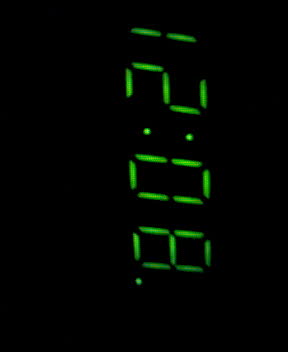The image depicts a black digital clock displayed in a close-up view, with the time "12:08" in bright green LED digits. The clock is oriented sideways, requiring a 90-degree turn to the left to read the time correctly. The numbers are slightly off-center, leaning more towards the right and the top of the black background. The time includes a colon between "12" and "08," and there is a small dot after the "08," which could indicate AM or PM. The digits are somewhat blurry and appear in a typical digital clock font, standing out starkly against the entirely black backdrop.